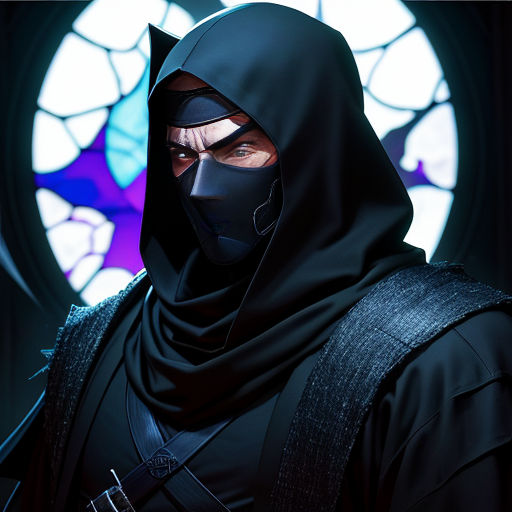This detailed drawing, styled as cartoon graphic art likely concept for a video game character, features a stern-looking man dressed in black attire, depicted from the chest up. His face is partially obscured by a Batman-like mask, complete with a pointy nose and black eyebrows framing his angry eyes. The character possibly embodies a samurai or ninja, with distinct features suggesting he's either a white or possibly an Asian man. His outfit includes a black shirt and crisscrossing leather belts over his chest, complemented by a black headband and a shadowy hood or scarf that adds to his mysterious appearance. On his left shoulder are prominent spikes and straps, enhancing his formidable aura.

The setting appears to be indoors, perhaps within a religious structure like a church, signified by a large, circular stained glass window in the background. This window displays a vivid array of colors, predominantly purples, blues, and white, with dark veins interwoven, contributing to the overall ominous ambiance of the scene. The dark, shadowy atmosphere of the setting accentuates the edgy, brooding nature of this enigmatic warrior.